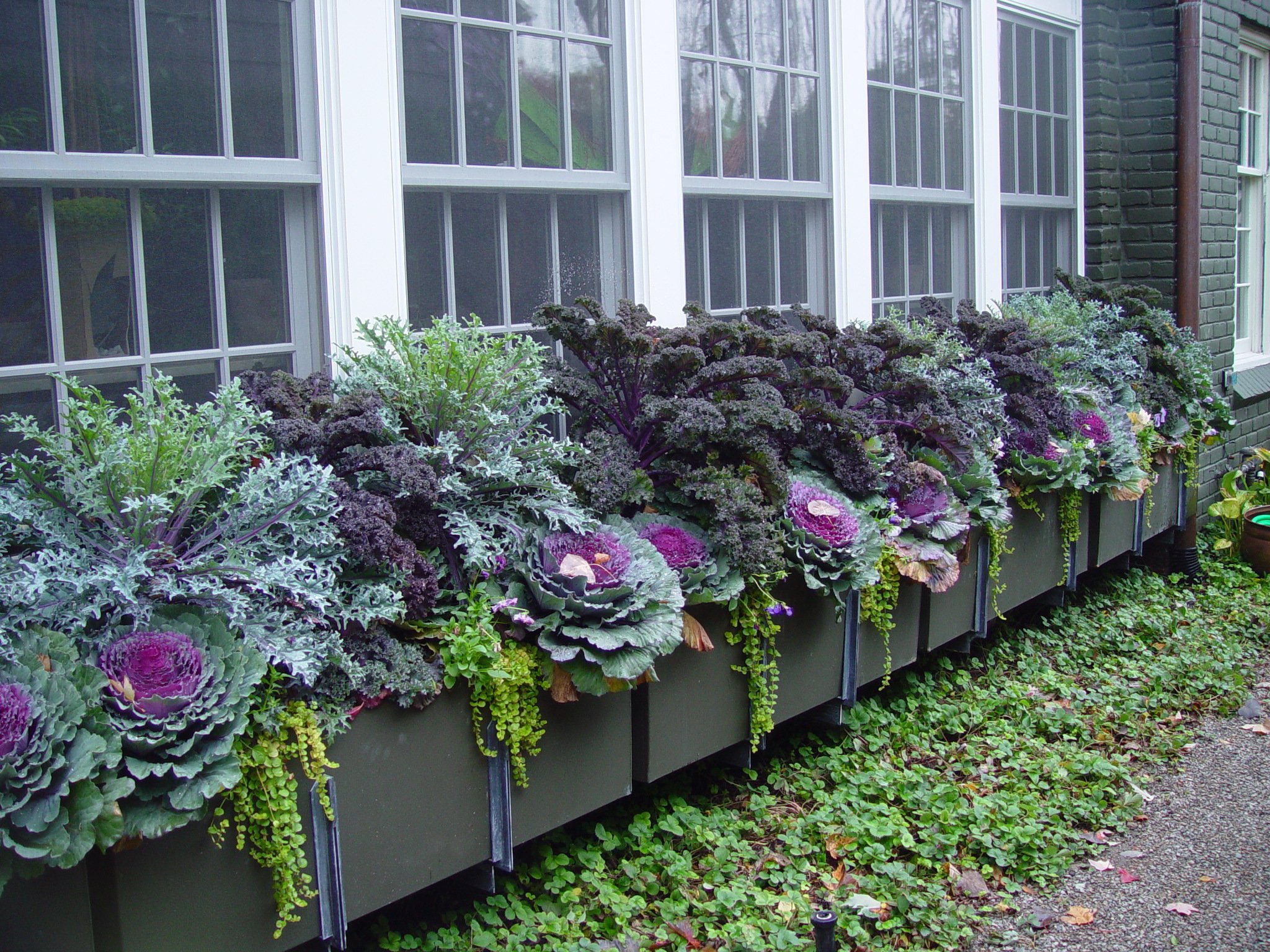This photograph captures the exterior of a dark gray brick building, taken outdoors during the daytime. The building's façade features five tall windows with white wooden trim, reflecting nearby trees. Below these windows, there are several long, gray plastic planter boxes filled with a variety of plants and flowers. The vibrant foliage displays an array of colors, including deep purple flowers, light green, mint green, and dark green leaves, some resembling kale or cabbage with purple centers. The planters are abundant, with some plants cascading over the sides. At the very bottom right corner, there is a gravelly walkway surrounded by a patch of clovers. The image also reveals the black head of a water sprinkler amidst the greenery.